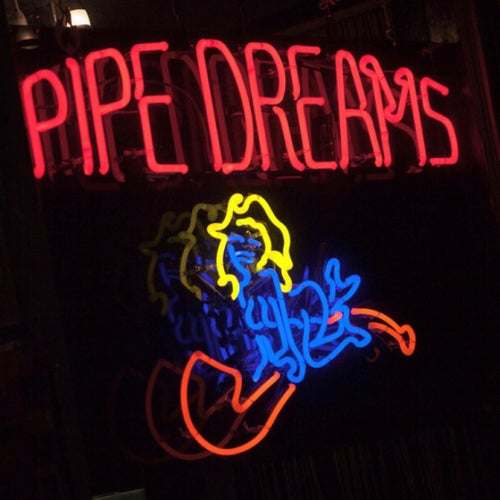The image features a striking neon sign set against a black background, accentuating its vibrant colors. At the top, the red neon lettering clearly reads "Pipe Dreams." Beneath the text, a vivid scene unfolds: a young, unclothed woman rendered in neon, her hair glowing yellow and her body outlined in blue. She is depicted in a kneeling position on her hands and knees, seemingly clinging to a red neon tobacco pipe. The entire composition, including the woman's detailed blue facial features and the red pipe, stands out distinctly against the dark backdrop, creating a bold and eye-catching display. A faint reflection suggests the sign might be in a window, possibly advertising a tobacco shop.